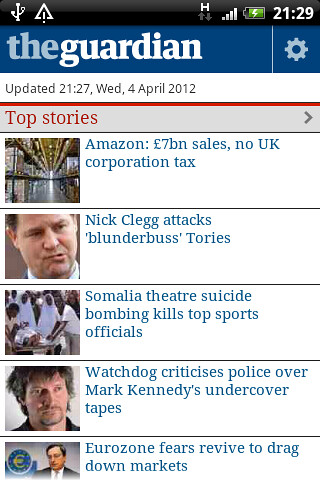The image is a screenshot displaying a selection of news articles from The Guardian. At the top, the title "The Guardian" is prominently featured, followed by an update timestamp that reads "Updated 21:27, Wednesday April 4th, 2012." Beneath this header, a series of headlines outline the top stories of the day, including:

1. "Amazon: £7 Million Sales, No UK Corporation Tax"
2. "Nick Clegg Attacks 'Blunderbuss' Tories"
3. "Somalia Theater Suicide Bombing Kills Top Sports Officials"
4. "Watchdog Criticizes Police Over Mark Kennedy's Undercover Tapes"
5. "Eurozone Fears: Survive to Drag Down Markets"

Each headline reflects significant events and issues, ranging from corporate tax controversies to international tragedies and economic concerns, capturing a broad spectrum of critical news topics.